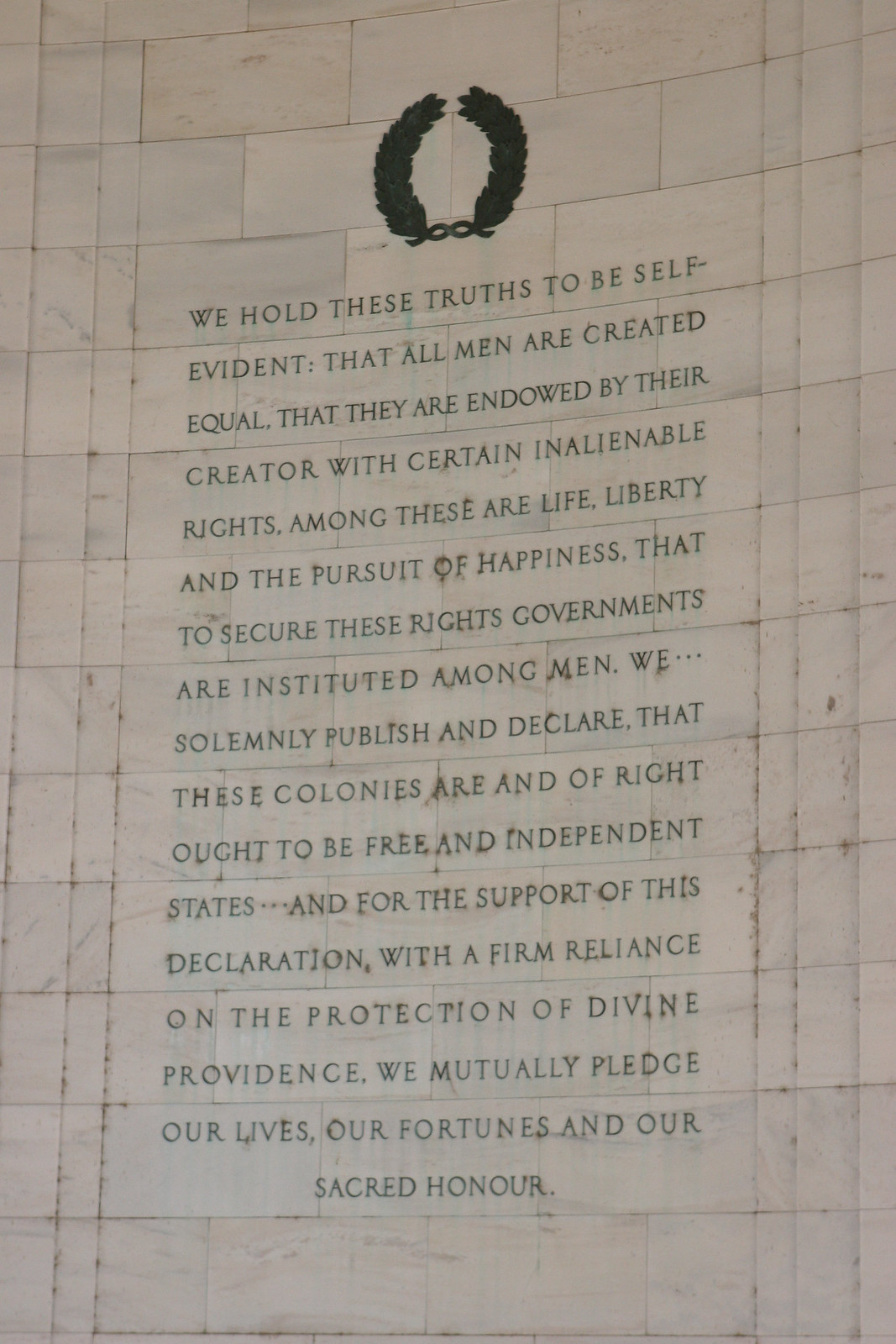The image depicts a detailed stone engraving on a tall, concave wall that appears to be made of marble or stone. A prominent black or dark green half-wreath emblem adorns the top of the structure. Below the emblem, inscribed in capital letters, is a profound excerpt: "We hold these truths to be self-evident, that all men are created equal, that they are endowed by their Creator with certain inalienable rights. Among these are life, liberty, and the pursuit of happiness. That to secure these rights, governments are instituted among men. We solemnly publish and declare that these colonies are, and of right, ought to be free and independent states. And for the support of this declaration, with a firm reliance on the protection of Divine Providence, we mutually pledge our lives, our fortunes, and our sacred honor." This inscription, reminiscent of the Declaration of Independence, appears to be a prominent feature at a historical site, potentially located in Washington, D.C. The structure's white or light-colored brick or stone wall provides a stark and reverent backdrop for the timeless words engraved upon it.